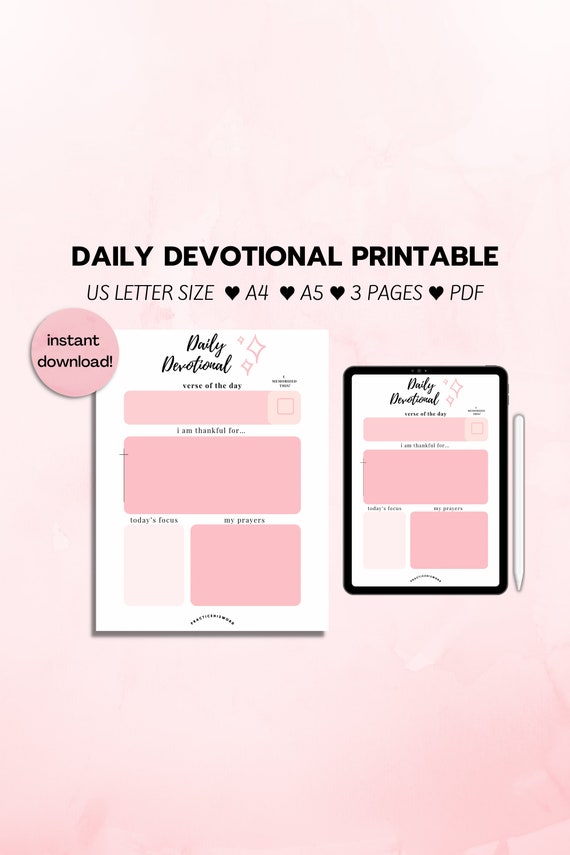The image depicts a listing for a daily devotional printable page, set against a pale pink background. The centerpiece is a photo of a daily devotional page, with black text reading "daily devotional" accompanied by small diamond shapes. Provided sections include "Verse of the Day" featuring a pink box intended for writing a verse, "I am Thankful For" where users can jot down things they are thankful for, "Today's Focus" in another pink box, and "My Prayers" with an additional space for notes. A pink circle on the page highlights "instant download," indicating easy accessibility. Adjacent to this image is a tablet or iPad showing the same devotional page, complemented by a white stylus. Above, bold black letters announce "Daily Devotional Printable," and additional details clarify it is available in US letter size, A4, and A5 formats, consisting of three pages in a PDF file.